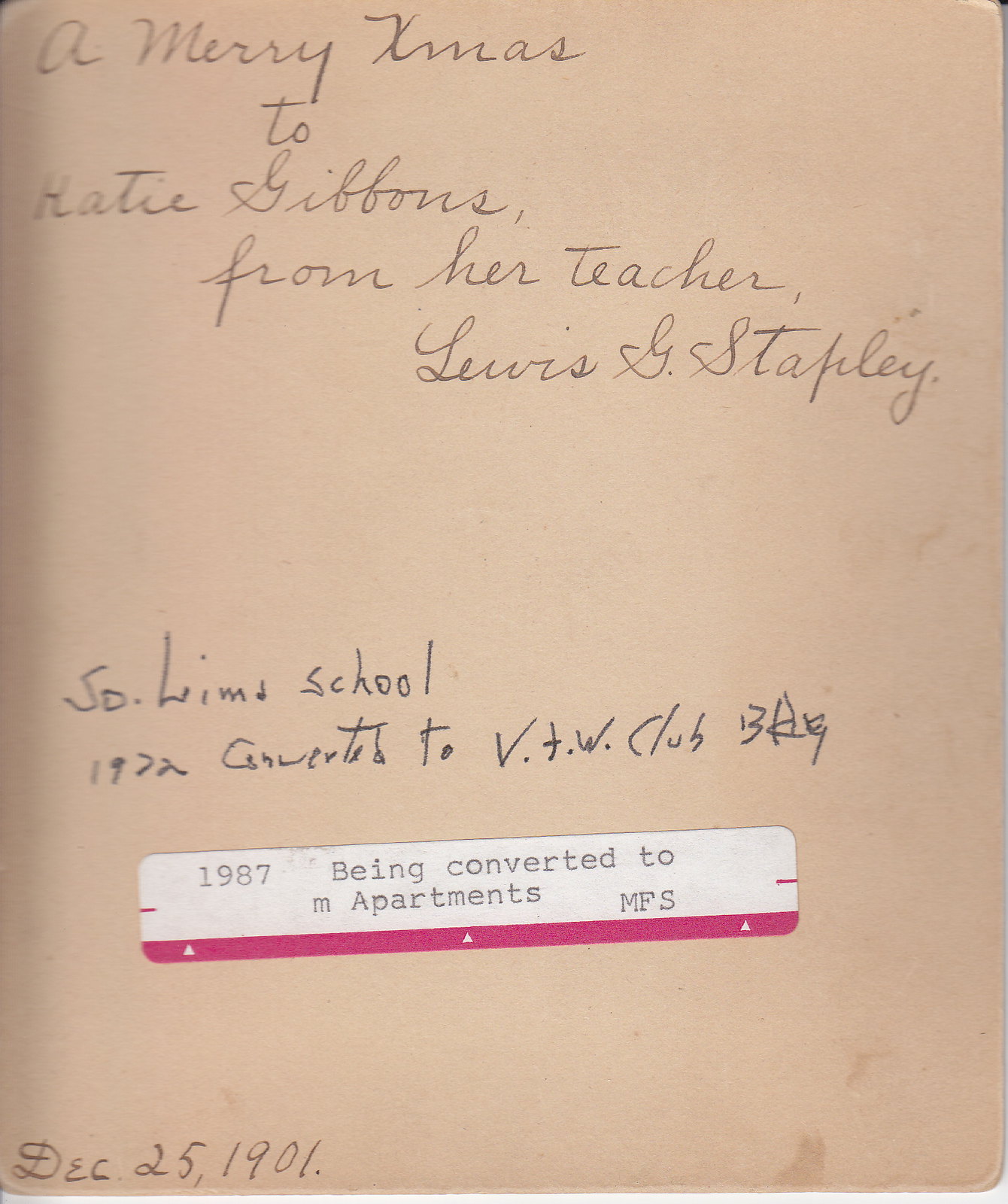The image depicts a discolored and stained handwritten letter on a piece of antiquated white paper. The text is written in cursive, likely with pencil or pen, and reads, "A Merry Xmas to Katie Gibbons from her teacher, Louis S. Stapley, South Lima School." The handwriting includes the date "December 25th, 1901" penned in old-fashioned ink in the bottom left-hand corner. The central lower portion of the paper bears a white label with a red border reading, "1987, being converted to M Apartments, MFS." Despite some illegible sections and variations in the recording, it appears the document has been updated over time, showing different dates and possibly addresses. The letter encapsulates a personal holiday greeting from 1901, later annotated and repurposed in 1987.